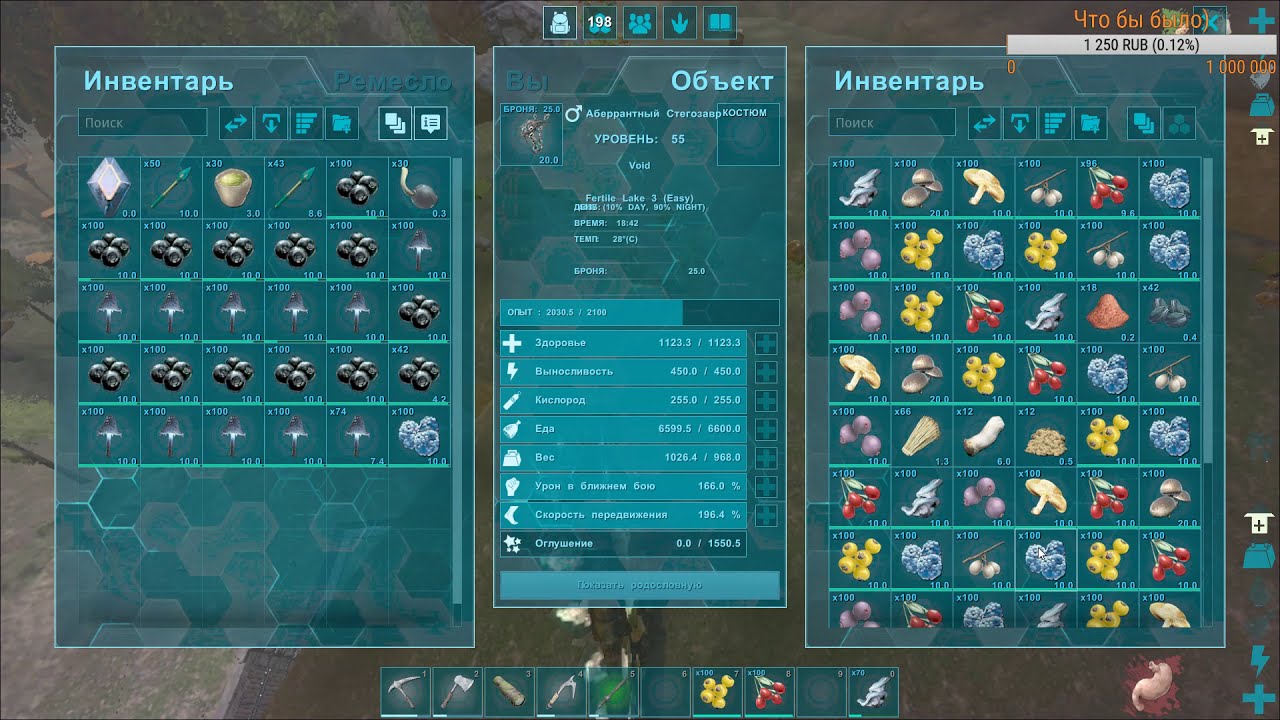The image is a screenshot of a Russian video game, indicated by the Cyrillic font and currency in rubles, suggesting an Eastern European setting. The central focus is on an inventory management system. On the right side of the screen, there is a grid of colorful items organized in rows of six by eight, primarily consisting of gathered resources such as wild fruits, berries, and mushrooms. The left side features a grid of predominantly gray or black items in rows of six by four, which appear to be tools and equipment like a pickaxe and a wood-cutting axe. The bottom section contains a rectangular toolbar displaying various tools and items necessary for tasks like mining and woodcutting, including logs or other resources. The background of the inventory screen is semi-transparent with a teal hue and hexagonal patterns, faintly revealing the outdoor environment of the game world behind it. The central display seems to feature a skills tree or character statistics, providing details on health, energy, and other attributes.